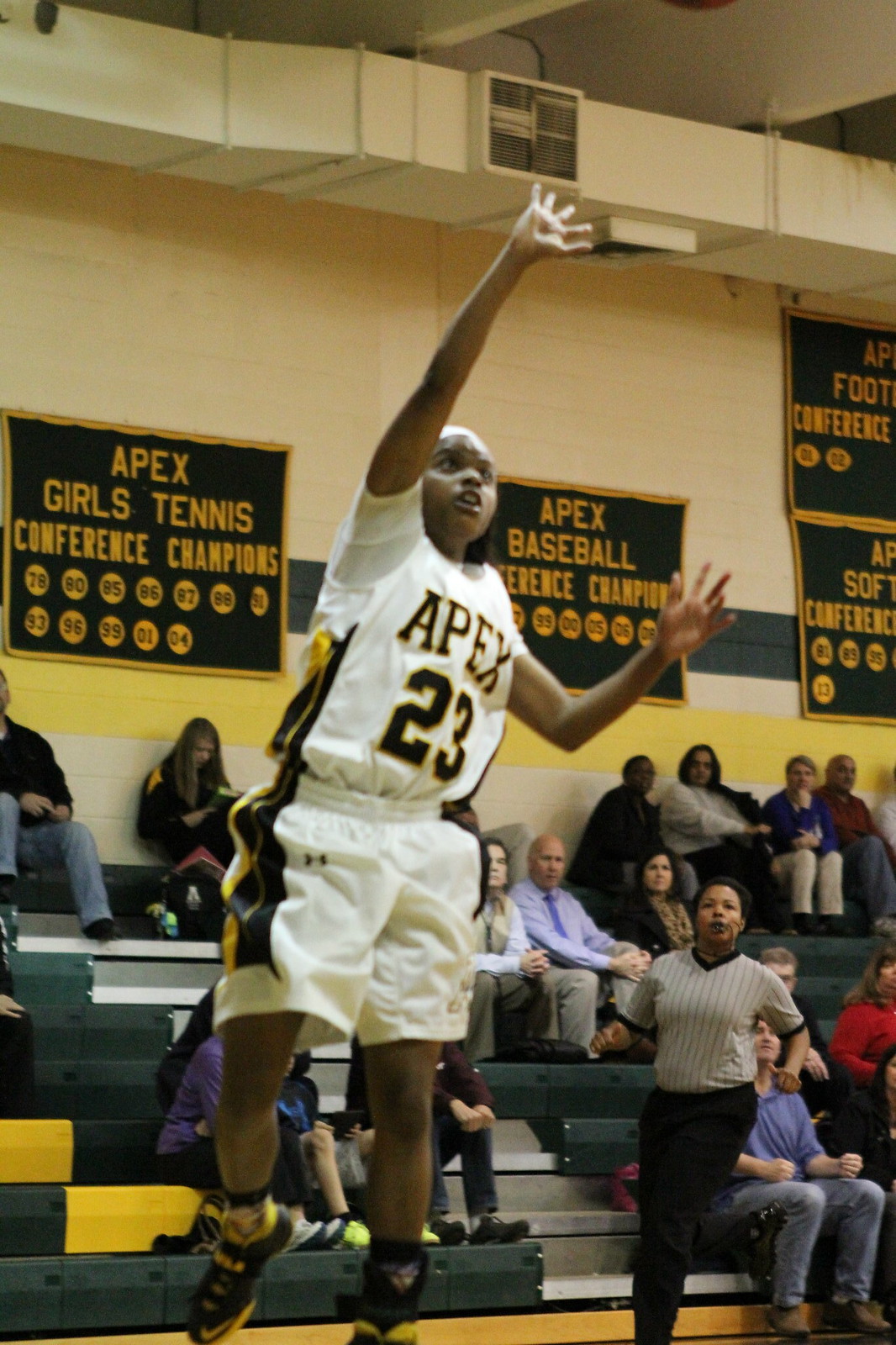An African American high school basketball player, wearing a white jersey with the number 23, white shorts, and blue and gold tennis shoes, is captured mid-air, possibly making a jump shot, though the basketball and hoop are not visible. He appears to be playing inside a gymnasium with green walls, where several banners hang. On the left wall, a yellow-on-black banner reads "Apex Girls Tennis Conference Champions" with dates listed below. To his right, another banner, partially readable, says "Apex Baseball Conference Champion." Further right, there are two more banners along the edge. In the background, bleachers are filled with spectators. An African American female referee, dressed in a striped jersey and dark pants, is running towards the player. The scene suggests a lively high school sports event, with the school's colors likely being gold and black.